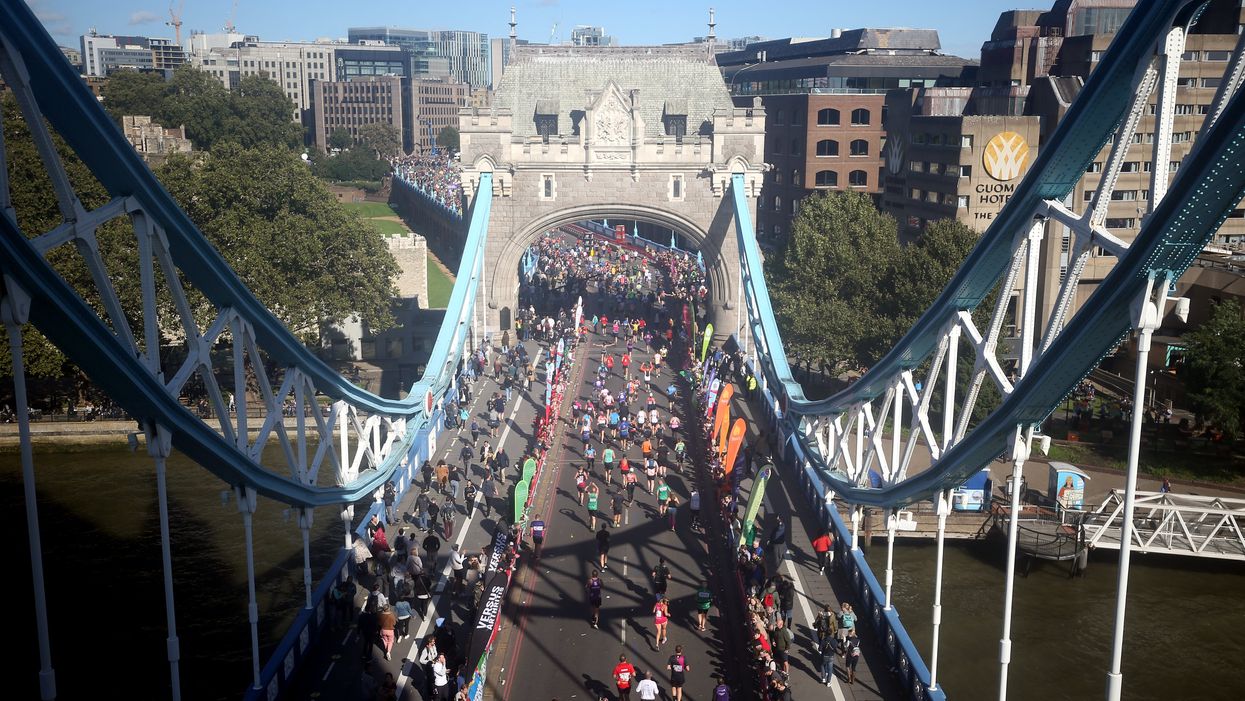The image depicts a semi-aerial, top-down view of a suspension bridge made of a blue metal frame, with a road passing through a large, castle-like stone archway reminiscent of medieval ramparts. The bridge, spanning over a body of water that leads to a cityscape, is filled with a massive crowd of colorful marathon runners. The runners, donning jerseys in various bright colors such as red, green, black, purple, and yellow, occupy the entire roadway, which is otherwise meant for vehicles. On either side of the cordoned-off area where the runners are, bystanders can be seen cheering and taking pictures. In the background, lush trees frame the scene, leading up to an expanse of towering gray and brown skyscrapers. Notably, a building labeled the Cuomo Hotel is visible on the right side of the image, providing a hint of the location. The marathon scene unfolds under daylight, capturing the vibrant spirit and communal energy of the event.